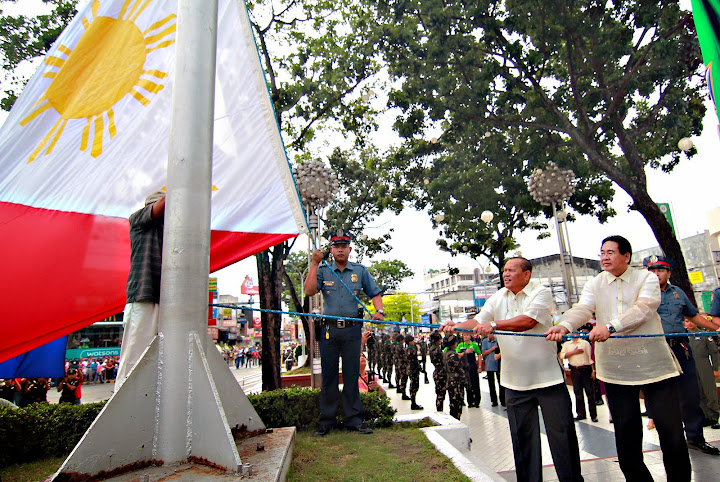In this outdoor photo of what appears to be a parade or ceremonial event, two men are prominently featured in the foreground on the right side. Both are dressed in collared white shirts, one with long sleeves and the other with short sleeves, and black pants. They are holding onto a blue rope that is connected to a tall, white rocket-like statue mounted on a small square cement platform. The rocket's top extends out of the frame, and next to it is a large flag. The flag, supported by the blue rope, features a white section with an image of a yellow sun and red on the other half, suggestive of the Philippines' flag. Another man, wearing white pants and a plaid shirt partially obscured by the statue, stands nearby. In the background, underneath a canopy of trees against a white sky, is a police officer dressed in a blue short-sleeved shirt and a hat, standing by the rope and monitoring the scene. On the sidewalk further back, a line of soldiers in uniform faces the street, and a large gathering of people fills the scene, indicating this is a significant outdoor event taking place in an urban setting.